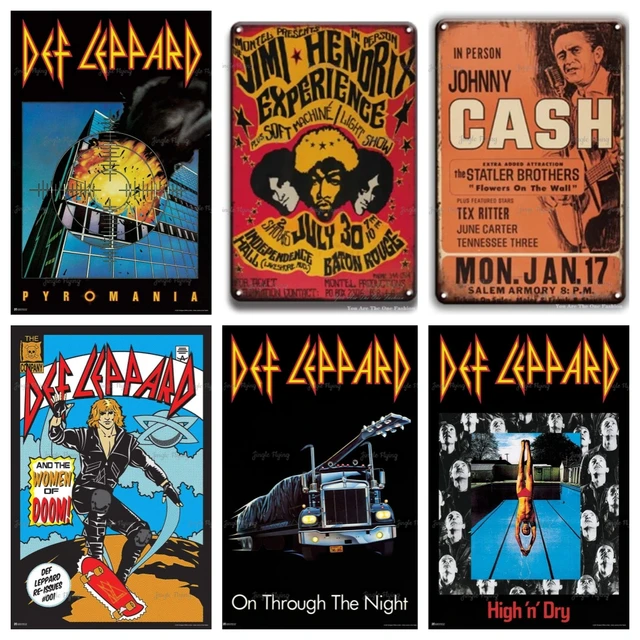A collection of six vintage concert posters, arranged in two rows of three, adorns the wall. In the top left corner, a Def Leppard "Pyromania" poster features crosshairs targeting a burning building. To the right, a vibrant red and yellow poster showcases the Jimi Hendrix Experience, listing a performance date of July 30th in Baton Rouge, with images of the band members’ heads mid-poster. The top right corner holds an orange poster advertising an in-person Johnny Cash concert, featuring a black-and-white portrait of Cash on a salmon-colored background. The bottom row exclusively displays Def Leppard posters: on the left, an animated man on a skateboard captioned "Def Leppard and the Women of Doom"; in the center, a semi-truck with an enormous guitar labeled "Def Leppard On Through the Night"; and on the right, a diver plunging into a pool stating "Def Leppard High and Dry." Each poster is slightly taller than it is wide, collectively creating a visually striking square of musical nostalgia.